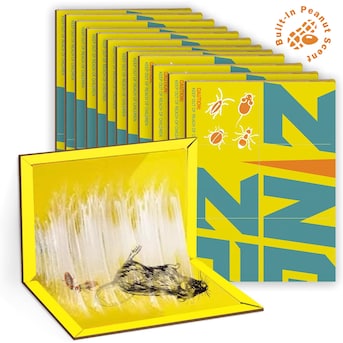This vibrant advertisement for rodent traps features an intricate illustration rather than a photograph. Dominated by bright yellow boards with bold blue and orange details, the image prominently displays a stack of traps, emphasizing their ample quantity, potentially indicating they come in packs of 14. The top left corner touts the product's "built-in peanut scent," accompanied by an image of a peanut, highlighting its irresistible appeal to pests.

The foreground presents an unsettlingly detailed open sticky trap, complete with a dead rat ensnared in a white adhesive mess, alongside several insects, including cockroaches and ants. The design of the trap resembles a three-dimensional card that can be closed, trapping the pests inside. The yellow boards are cluttered with images of various pests like ants, ticks, mice, and silverfish, reinforcing the trap's versatile effectiveness. Despite the vibrant colors, the grim depiction of pests trapped in the adhesive creates a disturbing yet compelling advertisement for this highly effective rodent trap.